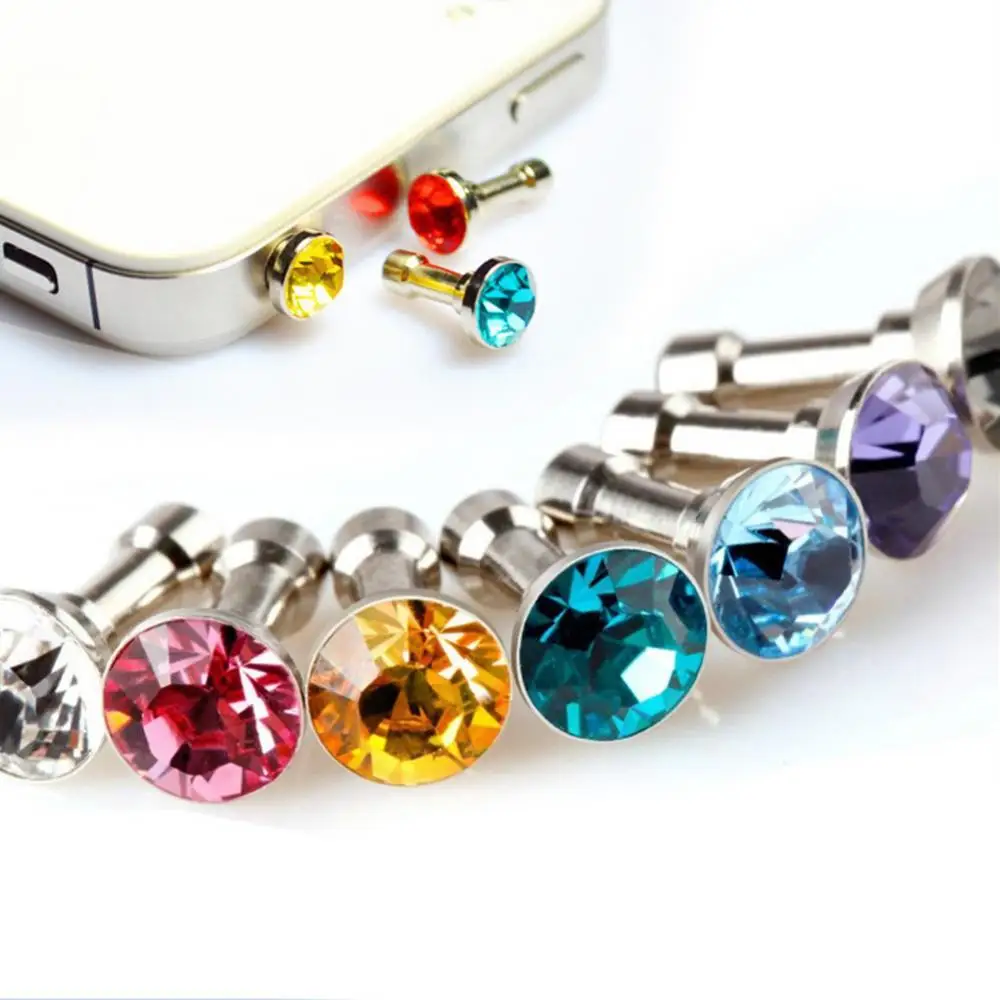The photograph showcases an assortment of gemstone-like emblems designed to be attached to headphone jacks. At the top of the image, part of an Android phone—likely an older model given the presence of a headphone jack—can be seen with a yellow emblem inserted into the socket. Surrounding the phone are various jewel emblems in a rainbow-like assortment, including white, pink, gold, teal, sapphire blue, amethyst purple, and reddish pink. These emblems are mounted on either silver or gold posts and are arranged in an orderly fashion against a white backdrop. In addition to the yellow emblem inserted into the phone, a red and a blue emblem are positioned nearby, further adding to the array of colorful gems decorating the scene. The entire composition is set against a clean, modern, and predominantly white background, highlighting the vivid colors of the jewels.